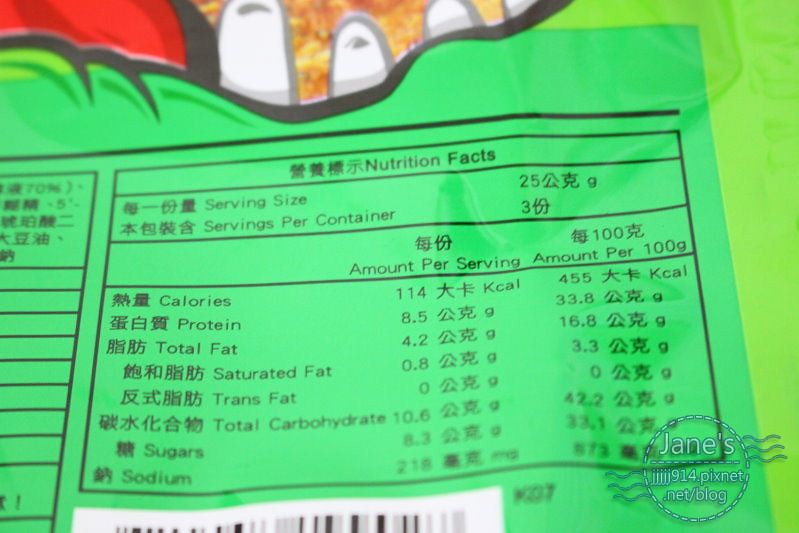The image depicts a predominantly green background which hosts a nutrition facts label in both English and an Asian language, suggesting the packaging originates from an Asian company. The top portion of the label is partially cut off, showing hints of red and white that resemble hands in a 3D effect, possibly intended to appear as if grasping the packaging. Below this image and to the left, there is a distinct black line that leads into the main section of the label, which lists detailed nutritional information per serving and per 100 grams: 114 and 455 calories, 8.5 and 33.8 grams of protein, 4.2 and 16.8 grams of total fat, 0.8 and 3.3 grams of saturated fat, 0 grams of trans fat for both measures, 10.6 and 42.2 grams of total carbohydrates, 8.3 and 33.1 grams of sugars, and 218 and 573 milligrams of sodium, respectively. At the bottom of this section, there is a barcode on a white label. Additionally, a watermark at the bottom right corner reads "James jjjjj914.pixnet.net forward slash blog."